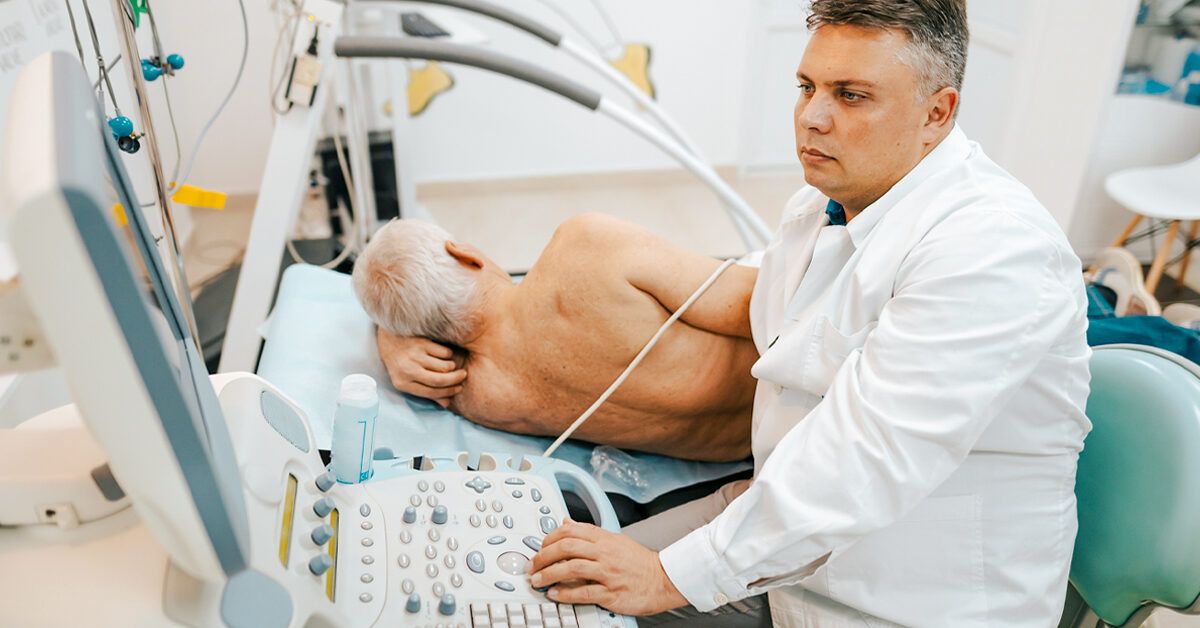This image depicts a detailed scene of a medical procedure in progress, likely involving the use of an ultrasound machine. At the center, a shirtless, gray-haired male patient with pale skin is lying on his left side on a hospital bed, his back to the camera. The patient has one arm positioned under his head. Seated to the left of the patient is a large, pale-skinned doctor (or technician) wearing a white lab coat. The doctor has close-cropped gray hair on the sides with darker hair on top. He is seated in a green swivel chair, facing a teal and white computer screen with teal buttons. The doctor's left hand operates the computer's control panel, while his right hand appears to be involved in the chest examination of the patient, possibly conducting a scan. The background includes an empty chair and open space, highlighting that these two individuals are the only ones present in the room.